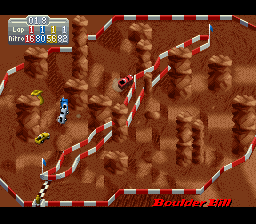This image is a screenshot of a video game titled "Boulder Hill." The game environment is characterized by numerous boulders dispersed throughout the scene. A red and white fence intricately weaves its way among the boulders, demarcating the inner area from the outer sections of the landscape. Within the gameplay screen, labels such as "Lop" and "Nitro" are visible, possibly indicating in-game options or power-ups. The scoreboard, set against a green background, displays scores in red, blue, yellow, and green. The players are represented by small blue and yellow vehicles that navigate over the boulders. A black and white checkered finish line signifies the goal, while the entire game screen is framed by black borders at the top and bottom.